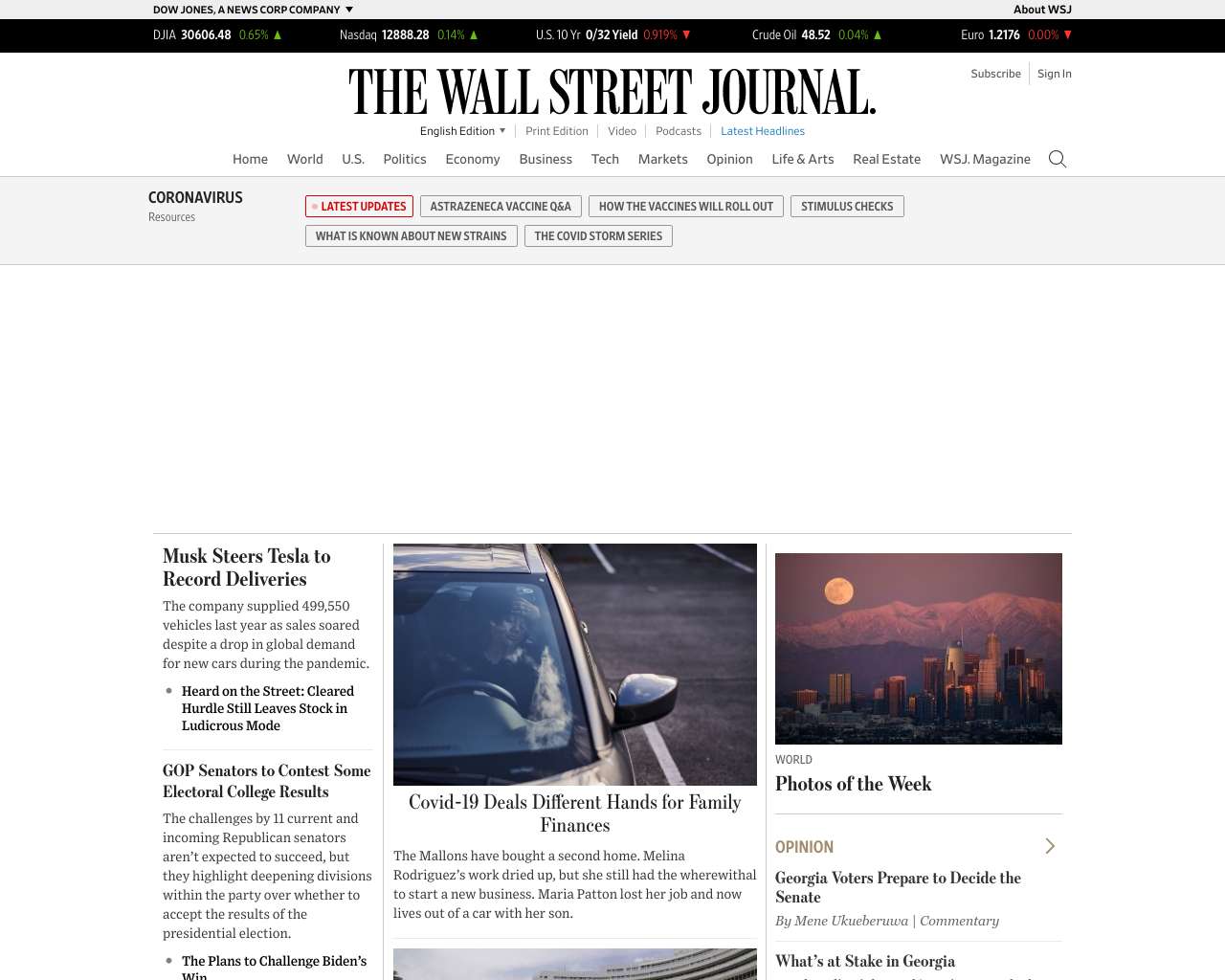**Caption:**

The image depicts a page from The Wall Street Journal website. At the top, the masthead displays "Dow Jones," denoting its affiliation with News Corp. Below this, the banner includes navigational options like "About WSJ," "Subscribe," "Sign In," and the selected "English Edition." Additional options such as "Print Edition," "Video," "Podcast," and a highlighted "Latest Headlines" in blue are also visible.

The primary navigation bar lists categories including "Home," "World," "U.S.," "Politics," "Economy," "Business," "Tech," "Markets," "Opinion," "Life & Arts," "Real Estate," and "WSJ Magazine." Just beneath these tabs, a section labeled "Coronavirus Resources" appears with "Latest Updates" highlighted in red.

Further down on the page are two featured photographs. The first image shows the driver's side of a car on a road, captioned "COVID-19 Deals Different Hands for Family Finances." The second photo depicts an urban landscape with a mountain and moon in the background, accompanying the header "World," and "Photos of the Week."

Among the story headlines displayed on the page, notable ones include "Musk Steers Tesla to Record Deliveries" and "GOP Senators to Contest Some Electoral College Results." Additionally, an "Opinion" section is featured with a headline "Georgia Voters Prepare to Decide the Senate," alongside related articles titled "What's at Stake in Georgia" and "The Plans to Challenge Biden's Win."